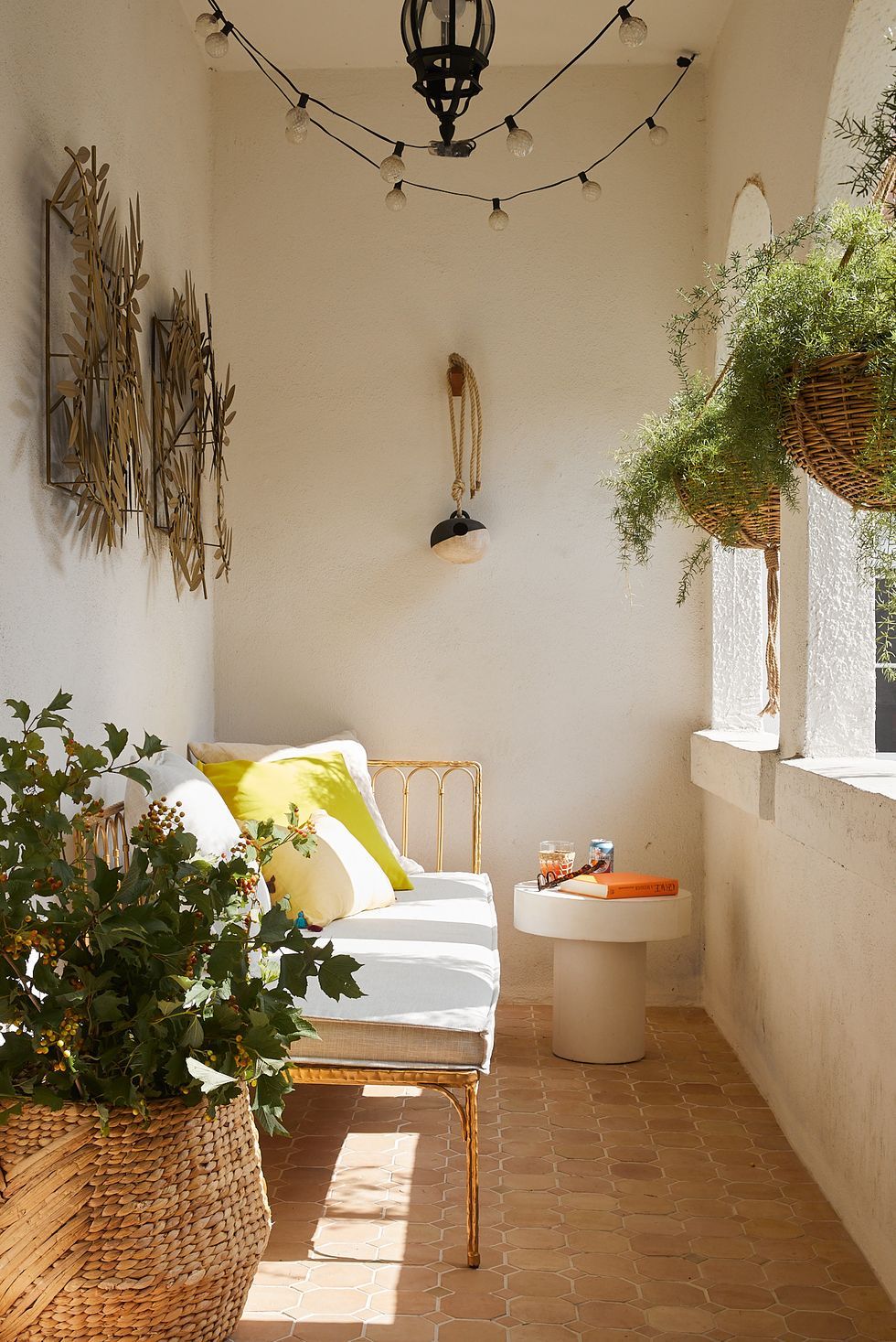The color photograph, taken in portrait orientation, depicts a small, narrow, and long covered terrace framed by three white walls. The space exudes a cozy yet stylish ambiance with its array of decor and furniture pieces. The terracotta-colored tiles with diamond patterns cover the floor, adding warmth to the setting. On the left side, a wicker settee couch, resembling a bed with a white mattress, is adorned with yellow and white throw pillows and features a metal frame. Above the settee hang two art pieces, side by side, showcasing bronze bamboo leaves on black square frames, contributing to an artistic touch.

A large wicker planter with a dark green plant stands beside the couch, closer to the viewer's left. In front of the settee is a mushroom-shaped small white table with an orange book placed on top. Two arched window openings on the right half wall provide a glimpse of the outdoors, each adorned with suspended brown wicker baskets from which green plants trail down elegantly. Overhead, two strands of Edison bulbs are suspended, casting a warm glow and adding to the intimate atmosphere.

In the upper right-hand corner, two more greenery-filled potted plants hang, enhancing the lushness of the terrace. Additionally, there is a hanging object on the wall in the background and two green wreaths adorn the left wall. This artistic and realistic photograph captures the terrace's inviting environment, characterized by its rustic elements and vibrant green plants.